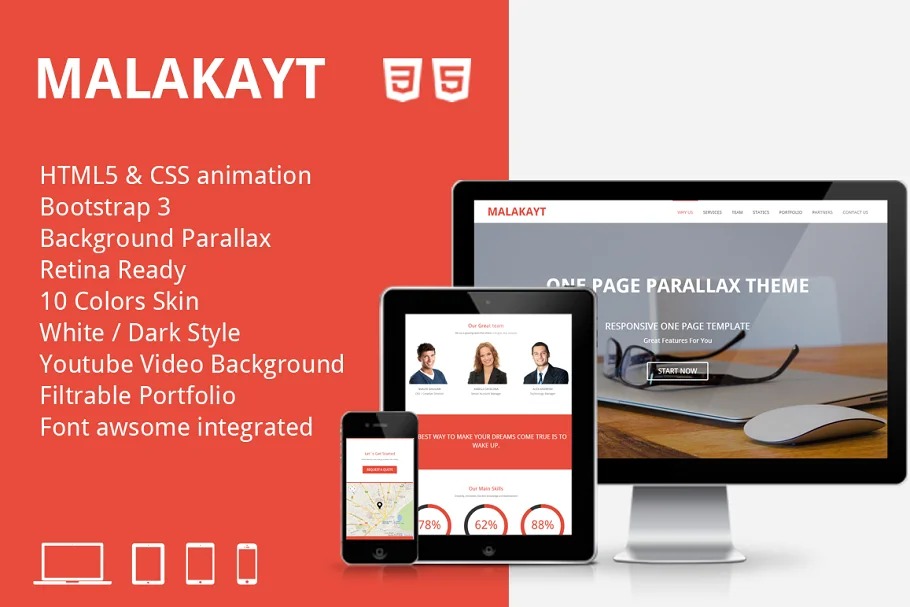The image is a display ad for a website theme, potentially a WordPress theme, though it doesn’t specify. The layout is rectangular, slightly wider than it is tall, almost square-like. The left half of the ad features a muted red background, while the right half has a very light gray, nearly silver background.

On the red side, the theme's name, "MALAKAYT," is prominently displayed in bold, white, capital letters. Adjacent to the name are two small white emblems resembling shields: one with a backward 'E' and the other with a stylized 'S.' Below these, there is a list of features and benefits written in white font against the red background. These features include:

- HTML5 and CSS animation
- Bootstrap 3
- Background parallax
- Retina ready
- 10 color skins
- White/Dark style
- YouTube video background
- Filterable portfolio
- Font Awesome integration

On the right side of the ad, there are three images showcasing the theme’s responsive design: one on a computer monitor, one on a tablet, and one on a mobile phone. These images demonstrate how the theme will appear on various devices, providing a visual representation of its adaptability.